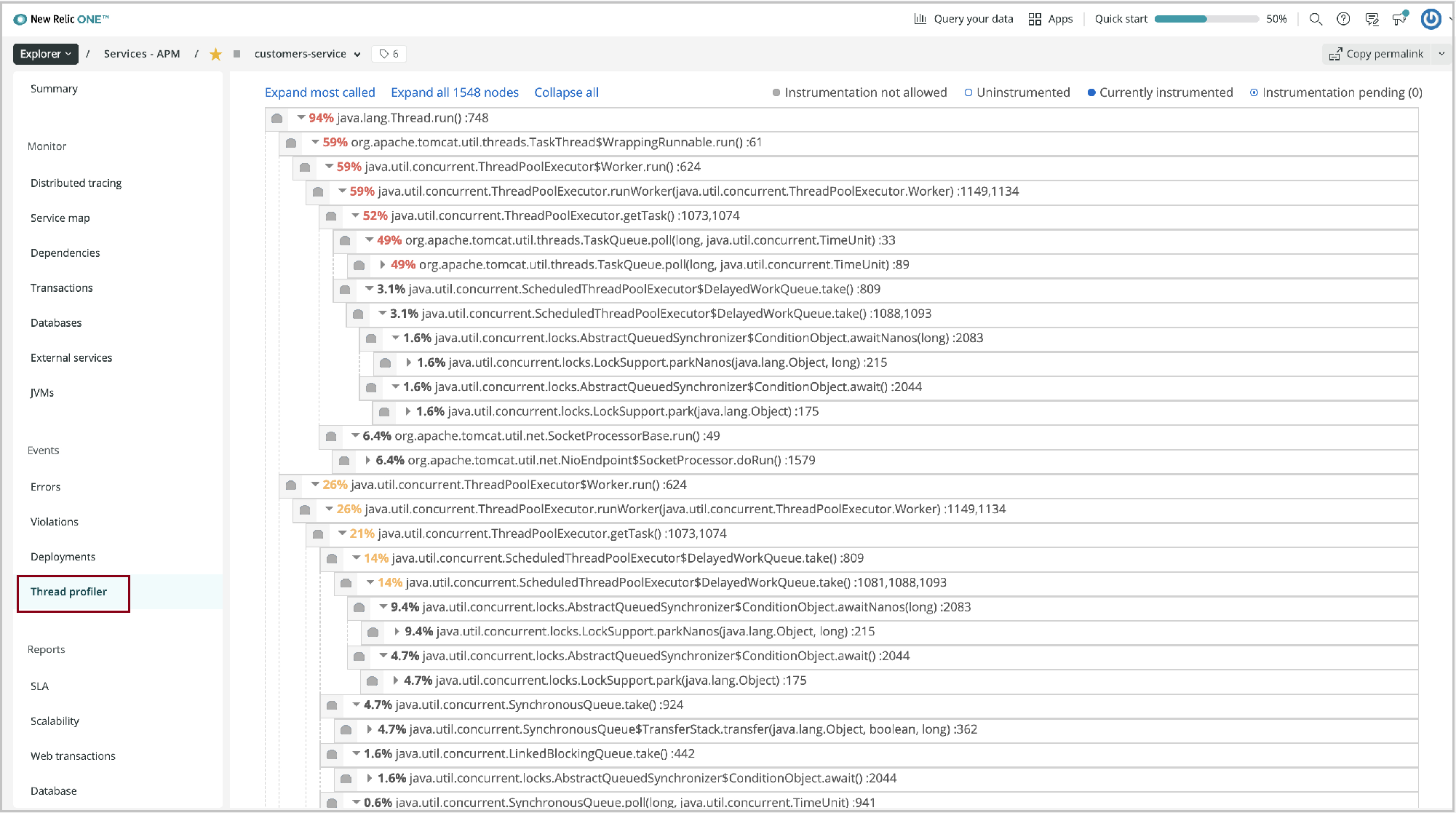Screenshot depicting a list with a white background, featuring detailed instrumentation statuses and percentages across various websites. The interface displays expandable options with "expand all" and "collapse all" buttons, alongside a total of 1,548 notes. The list categorizes items into the following sections: "Instrumentation Not Allowed," "Un-Instrumented," "Currently Instrumented," and "Instrumentation Pending" (the latter showing zero entries). The percentages representing different levels of instrumentation coverage across various websites are detailed as follows: 
- 94% on one website,
- 50% on another,
- 59% on a third,
- 3.1% on a fourth,
- 1.6% repeated on three sites,
- 6.4% on the last listed website.